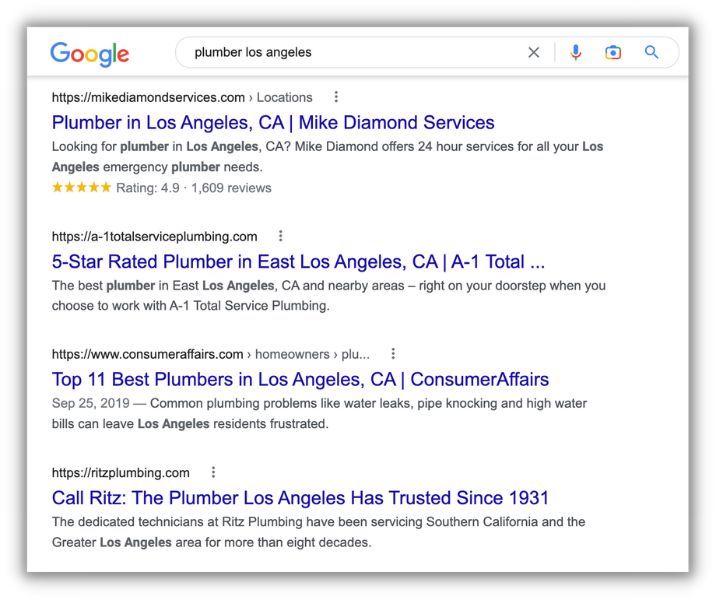The image is a rectangular landscape screenshot of a Google search results page, marginally wider than it is tall by about 10%. The entire background is white with a thin shadow around all sides, creating a slightly popped-out effect. 

At the top 10% of the image is the Google header strip. In the upper left corner is the Google logo in its standard multi-colored font. To the right is the long, stretched-out search bar with rounded corners. The search query "plumber los angeles" is entered in lowercase, left-justified text. At the far right of the search bar, there is a gray "X" icon, a vertical gray line, followed by three color icons: a microphone, a camera, and a magnifying glass.

Below the search bar, four search results are displayed, each following a similar format:

1. **First Result:**
   - **Web Address:** `https://www.mikediamondservices.com`
   - **Details:** Next to the web address, there is a rightward-facing arrowhead followed by the label "locations" in gray and three vertical gray dots.
   - **Title:** "Plumber in Los Angeles, CA" in larger blue font.
   - **Source:** "Mike Diamond Services" in blue font, separated by a vertical line.
   - **Description:** One and a half lines of smaller gray text beginning with "Looking for Plumber in Los Angeles, CA?" Both "Plumber" and "Los Angeles" are bold.
   - **Rating:** Five yellow-orange stars with the text "Rating: 4.9 – 1,609 reviews" to the right.

2. **Second Result:**
   - **Web Address:** `https://www.a1totalserviceplumbing.com`
   - **Details:** This result does not have a "locations" callout.
   - **Title:** "5-star rated plumber in East Los Angeles, CA" in larger blue font.
   - **Source:** "A-1 Total..." in blue font, following a vertical line.
   - **Description:** One and a half lines of smaller gray text beginning with "The best plumber in East Los Angeles, CA." "Plumber" and "Los Angeles" are bold.
   - **Rating:** No rating stars or additional info provided.

3. **Third Result:**
   - **Web Address:** `https://www.consumeraffairs.com`
   - **Title:** "Top 11 best plumbers in Los Angeles, CA" in larger blue font.
   - **Source:** "Consumer Affairs" in blue font, with an initialism "CA" capitalized.
   - **Details:** One and a half lines of smaller gray text mentioning "SEP 25, 2019" followed by an em dash and more content, beginning with "common plumbing problems like water leaks."

4. **Fourth Result:**
   - **Web Address:** `https://www.ritzplumbing.com`
   - **Title:** "Call Ritz: the plumber Los Angeles has trusted since 1931" in larger blue font.
   - **Source:** Details below the title begin with "The dedicated technicians at Ritz Plumbing have been servicing Southern California," extending for one and a half lines.
   - **Rating:** No rating or additional info provided.

Each result includes three vertical gray dots aligning with the right edge of the list.